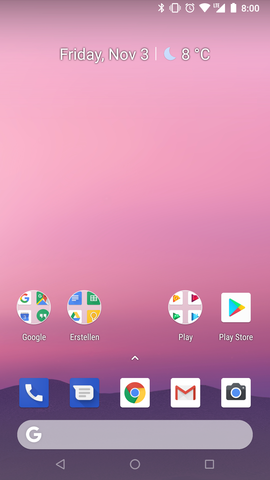A detailed screenshot of a phone's homepage features a minimalist layout. At the top of the screen, the status bar displays the current date, "Friday, November 3," alongside a crescent moon icon indicating nighttime. The temperature is shown as 8 degrees Celsius.

The home screen contains only a few essential apps, organized into two rows near the bottom. In the top row, from left to right, are the Google search bar, an app named "Airstellan," the Google Play app, and the Play Store icon. The bottom row holds five key applications: the phone's call app, messaging app, Google Chrome browser, Gmail, and a photo gallery app.

The background wallpaper showcases a striking image of a pink sky and purple mountains, adding a serene, colorful aesthetic to the minimalistic app arrangement. A Google search bar is prominently positioned at the bottom of the screen, providing quick access to the search function.